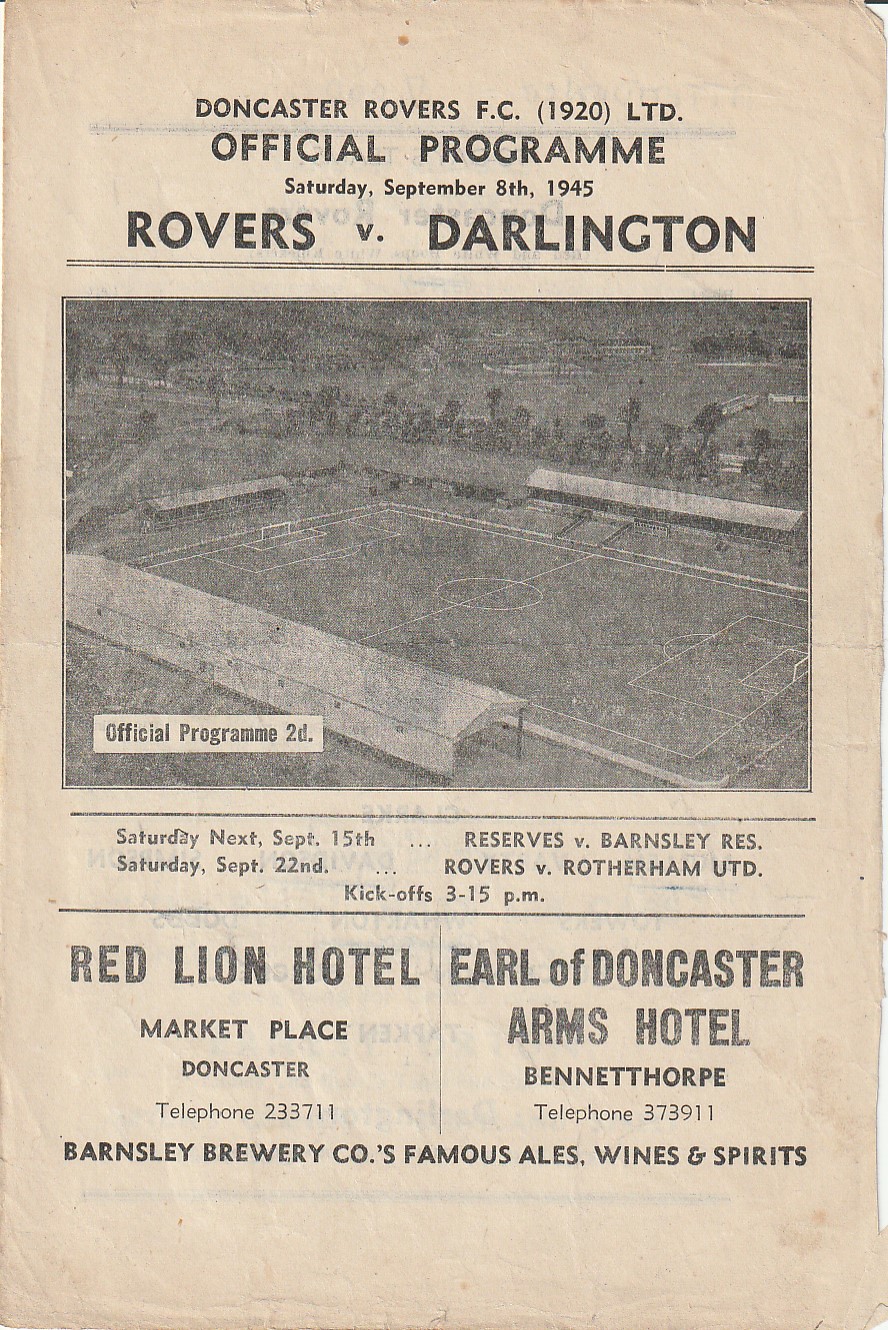This image is a scan of an official program for a soccer game between Doncaster Rovers and Darlington, dated Saturday, September 8th, 1945. The program is printed on aged, brown paper, so thin you can faintly see text from the other side. The header features "Doncaster Rovers FC 1920 Ltd Official Program" in black writing. Beneath this, a large black-and-white photograph or illustration showcases a soccer pitch with covered seating surrounding it and trees and houses in the background. The program is priced at 2D, a pre-decimal British currency. Below the main event, it lists upcoming matches: "Saturday Next September 15th, Reserves vs Barnsley Res," and "Saturday September 22nd, Rovers vs Rotherham UTD," both with kickoffs at 3:15 p.m. Mentioned sponsors include the Red Lion Hotel, Marketplace, Doncaster (Telephone 233711), and the Earl of Doncaster Arms Hotel, Bennetthorpe (Telephone 373911). At the bottom, there is a line promoting "Barnsley Brewery Company's Famous Ales, Wines, and Spirits."